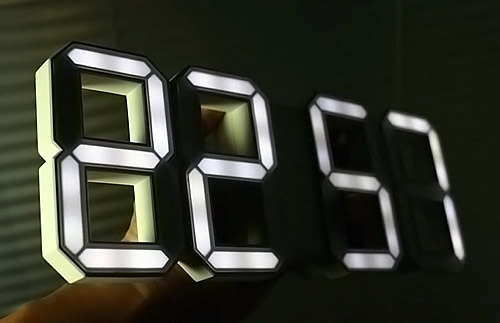In this image, we see a highly distinctive digital clock displaying the time 22:57 (or 11:57 PM for those not using the 24-hour format). The clock features an innovative design where the digits are rendered in three-dimensional segments. These segments can dynamically morph to form any numeral, making the entire clock face composed of adaptable 3D "blocks." The digits are primarily illuminated in white, while the unnecessary portions of the segments turn black, effectively creating the correct figures for the current time. This enables the clock to seamlessly transition between different times by simply altering which segments are visible. The clever design allows for a modern, sleek aesthetic while maintaining full functionality.